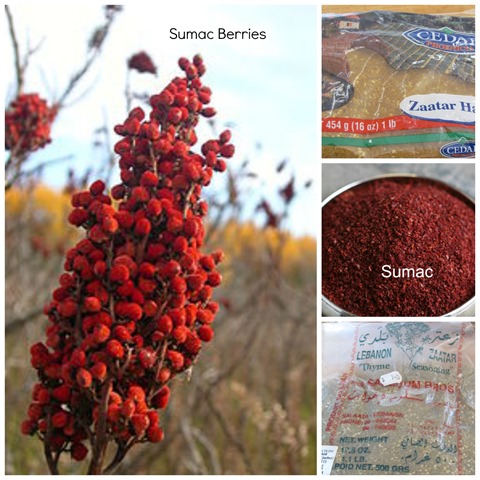The image is a collage of four photographs arranged in two main sections: one large photograph on the left and three smaller stacked photographs on the right. The large photograph to the left features a close-up of a stalk with clusters of red sumac berries against a blurred background of green grass and other plants, identified by the text "Sumac Berries" in the upper right corner. 

On the top right, a photograph shows a beige food product in a plastic package labeled "454 grams, 16 ounces, 1 pound," with additional readable text including "Z-A-A-T-A-R" and "cedar." The middle right photograph displays a bowl filled with red ground sumac, labeled "Sumac" in white text at the bottom. The bottom right photograph shows another plastic package containing a food product with labels, including "Lebanon" and "Z-A-A-T-A-R Thyme Seasoning."

The images are set against a blue, white, black, red, yellow, and green color palette, possibly as part of a product description or a comparative display of sumac-based items.